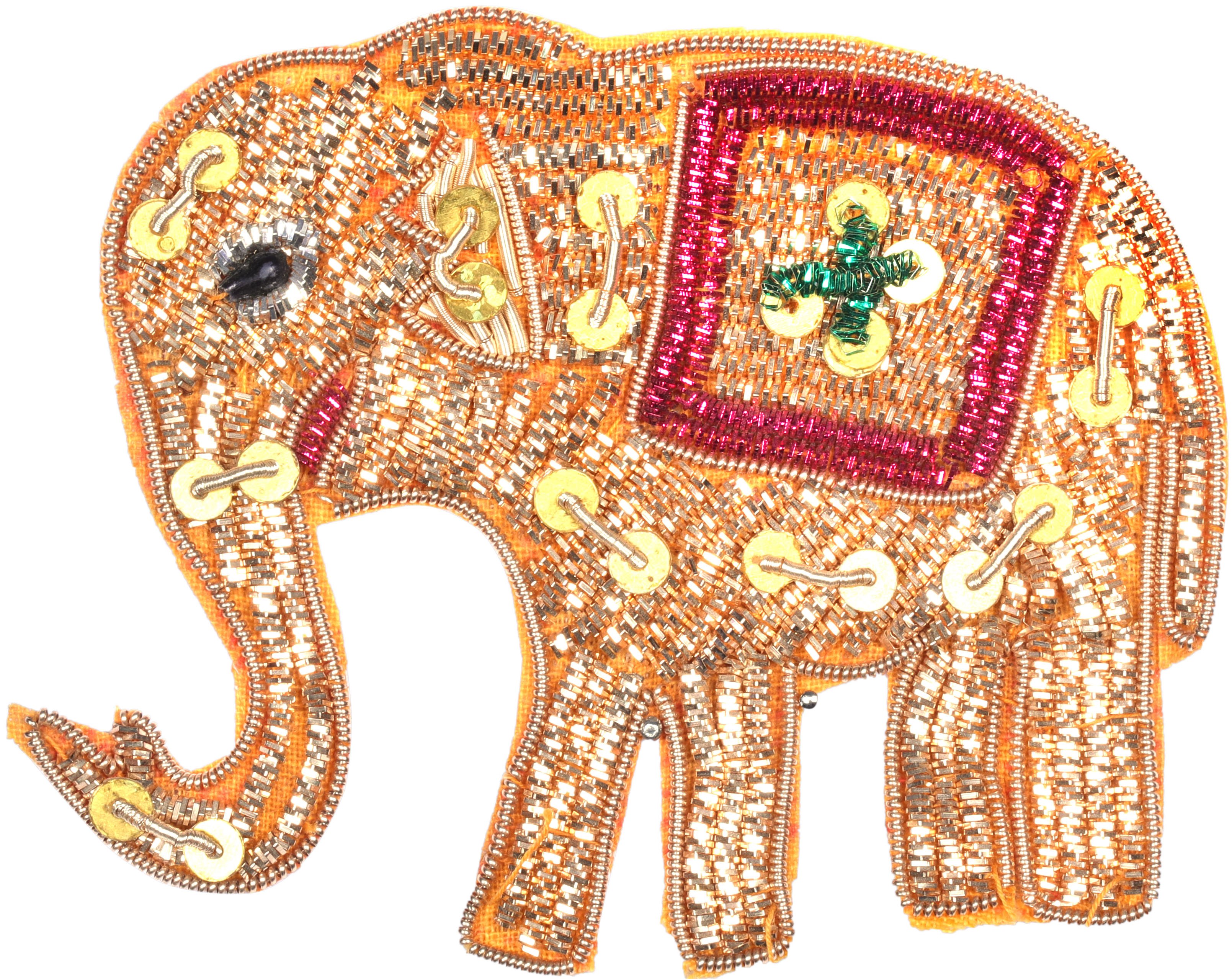The image depicts a large, flat, artistically crafted piece shaped like an elephant facing left, resembling a beaded or embroidered work, possibly crafted from orange fabric. The body of the elephant features intricate detailing with silver beads or thread lining its edges. The primary color of the elephant is orange with sections decorated using a combination of white, silver, and black beads arranged in various patterns. Scattered throughout its body are pale yellow circular elements, each connected by a horizontal piece of silver string; notable positions include the trunk, forehead, mouth, middle, and near the tail. The elephant's black eye contrasts sharply against its vibrant body. Draped across its back is a red blanket-like pattern, bordered by two red lines with white stitching, and adorned with a distinctive orange X in the center. This blanket design includes two green coiled shapes crossing each other. The overall background of the photograph is plain white, emphasizing the detailed and colorful craftsmanship of the elephant without any additional elements like text or people.